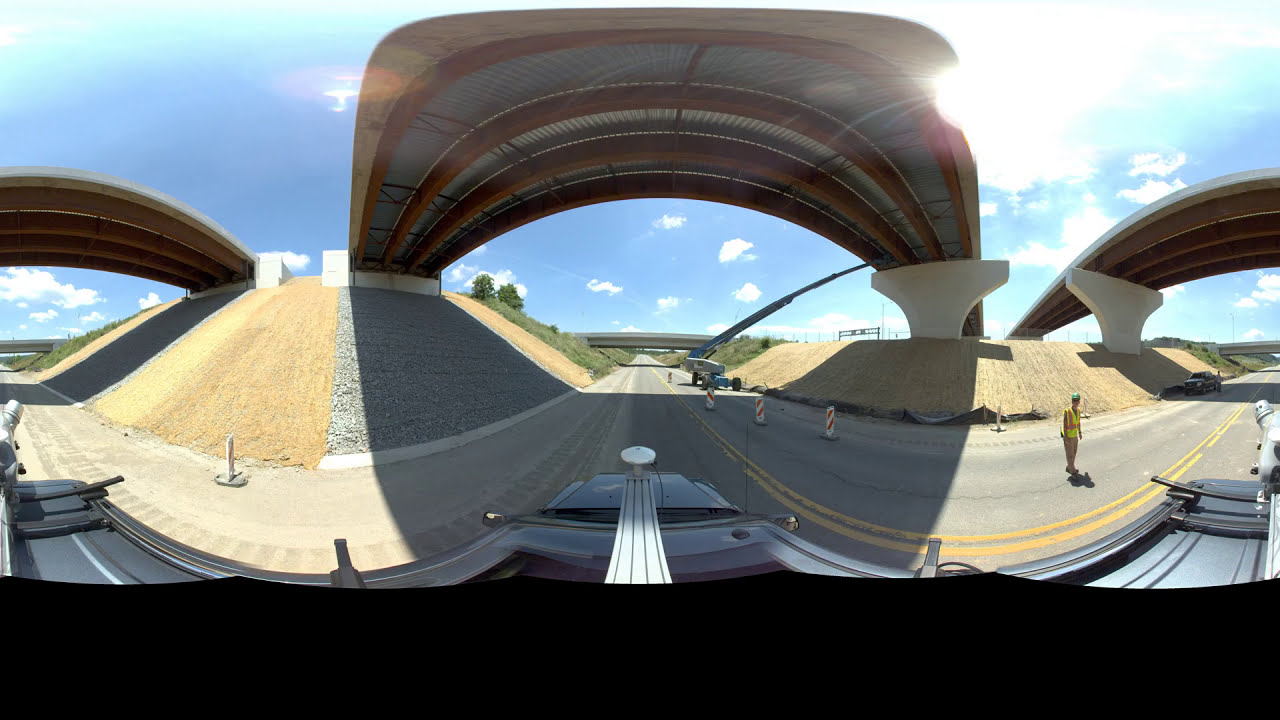This dynamic exterior daylight photograph, taken with a fisheye lens from atop a vehicle, depicts a vibrant construction scene under a bridge. The curvature from the lens distorts the view, making the bridge and surrounding structures appear curved and elongated. Ahead, a flat gray asphalt road with double yellow lines stretches out, bordered by brown walls and a white column supporting the overpass. Orange and white traffic cones delineate the closed-off right side of the road, where a worker stands in a yellow and orange reflective vest, khaki pants, and a blue helmet. Off in the distance, a tall blue and white crane is actively engaged in work on the overpass. The bright, partly cloudy sky with small, patchy clouds adds to the vividness of the scene, framed by patches of green trees and grass. The bright sun enhances the clarity and vibrancy of the construction zone, bringing out the details and colors of the bustling activity.